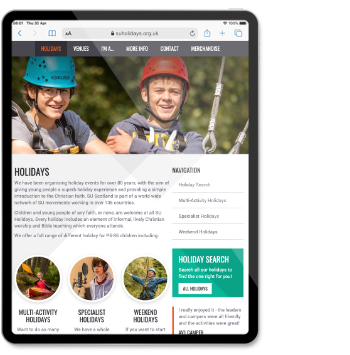The image depicts a blurry, zoomed-out screenshot of a web browser, likely Safari, shown on a tablet. The top section of the browser includes a gray search bar with navigation controls—a blue-highlighted "Back" button and a grayed-out "Forward" button—indicating that forward navigation is not currently available. Additionally, there's a blue history option, a greyed-out URL field, and several interactive icons to the right, including refresh, share, add, and an unidentified option with overlapping boxes.

The main part of the image appears to be an advertisement promoting holiday activities. The top of the ad features six clickable options, with the current selection highlighted in orange, while the remaining options are in white font. The central focus of the ad is a photograph showing a young girl and boy wearing helmets, possibly preparing for a zip-lining activity. Large black font prominently displays the word "Holidays," emphasizing the theme of the advertisement. Despite the overall blur of the image, the theme and elements convey a sense of adventure and holiday fun.